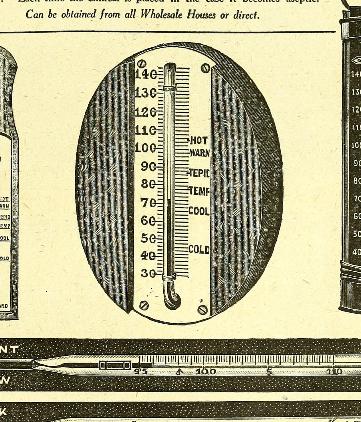This detailed illustration appears to be from an old-fashioned manual. The image has a faded yellowish background, giving it a nostalgic and aged look. The main graphic is rendered in black and white with a grainy texture that adds to its vintage feel. At the top of the image, partial text is visible, stating, "can be obtained from all wholesale houses or direct."

Below this text is a circular illustration of a thermometer. The thermometer is marked with temperatures ranging from 140°F at the top to 30°F at the bottom. Along the side of the thermometer, qualitative temperature labels are present: "hot," "warm," "temp," "cool," and "cold."

Flanking either side of this central illustration are partial views of additional black and white graphics, whose details are obscured. At the bottom of the image, a long rectangular object is visible, featuring some black text and numbers, further emphasizing the instructional nature of the illustration.